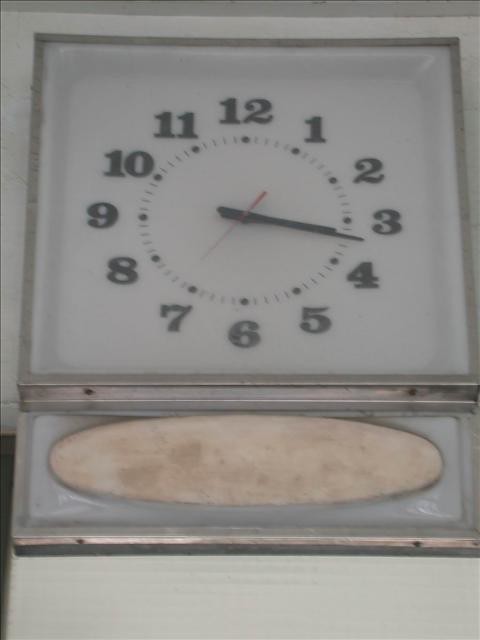This image features a detailed close-up of an antique wall clock, prominently framed in silver metal. The clock's face is a crisp, clean white, contrasted by its bold black numerals for easy readability. Both the hour and minute hands are slender and black, while the second hand is distinctly red, adding a striking detail. Minute increments are denoted by small black dots beneath each number. Below the clock face, there is a rectangular attachment with an oval cut-out, though its exact function remains unclear. The clock's overall vintage aesthetic suggests it is an older model, exuding a timeless, classic charm.